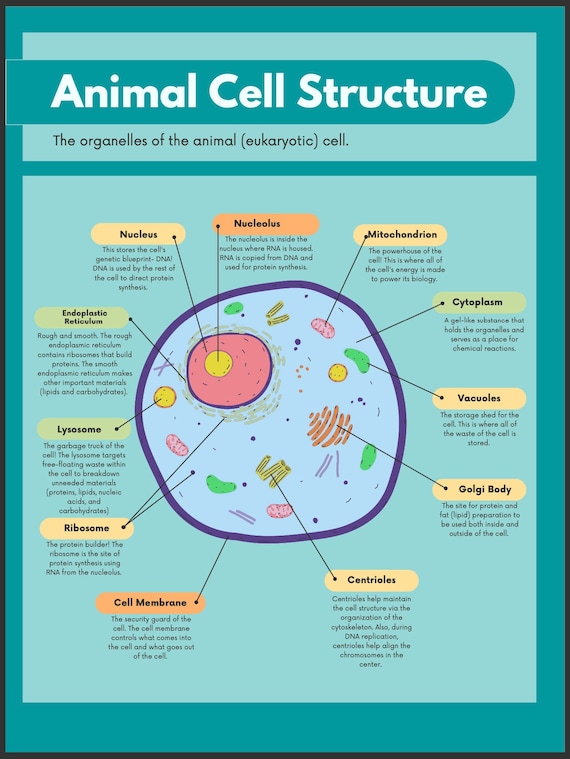This image is a highly detailed poster illustrating the structure of an animal cell, typically used for educational purposes, such as a science lesson. At the top of the poster, a turquoise blue outer barrier contains a banner that reads "Animal Cell Structure" in white letters on a dark teal blue background. Just below this, another label explains, "The organelles of the animal eukaryotic cell."

The central part of the poster features a round diagram of the cell, outlined in dark purple with a lighter purple interior. The cell houses a large pink nucleus, which contains a yellow nucleolus. Various organelles within the cell, including the mitochondria, cytoplasm, vacuoles, Golgi body, centrioles, cell membrane, ribosomes, lysosomes, and endoplasmic reticulum, are depicted in different colors for easy identification. Each organelle is connected to a label via a black line, providing brief descriptions of their functions.

The background of the poster transitions from a lighter blue in the center to a green gradient with an aqua blue perimeter and a black outer lining, enhancing the visual appeal and readability. This detailed and colorful representation makes it easy to follow and understand the components of an animal cell, serving as a valuable learning tool.